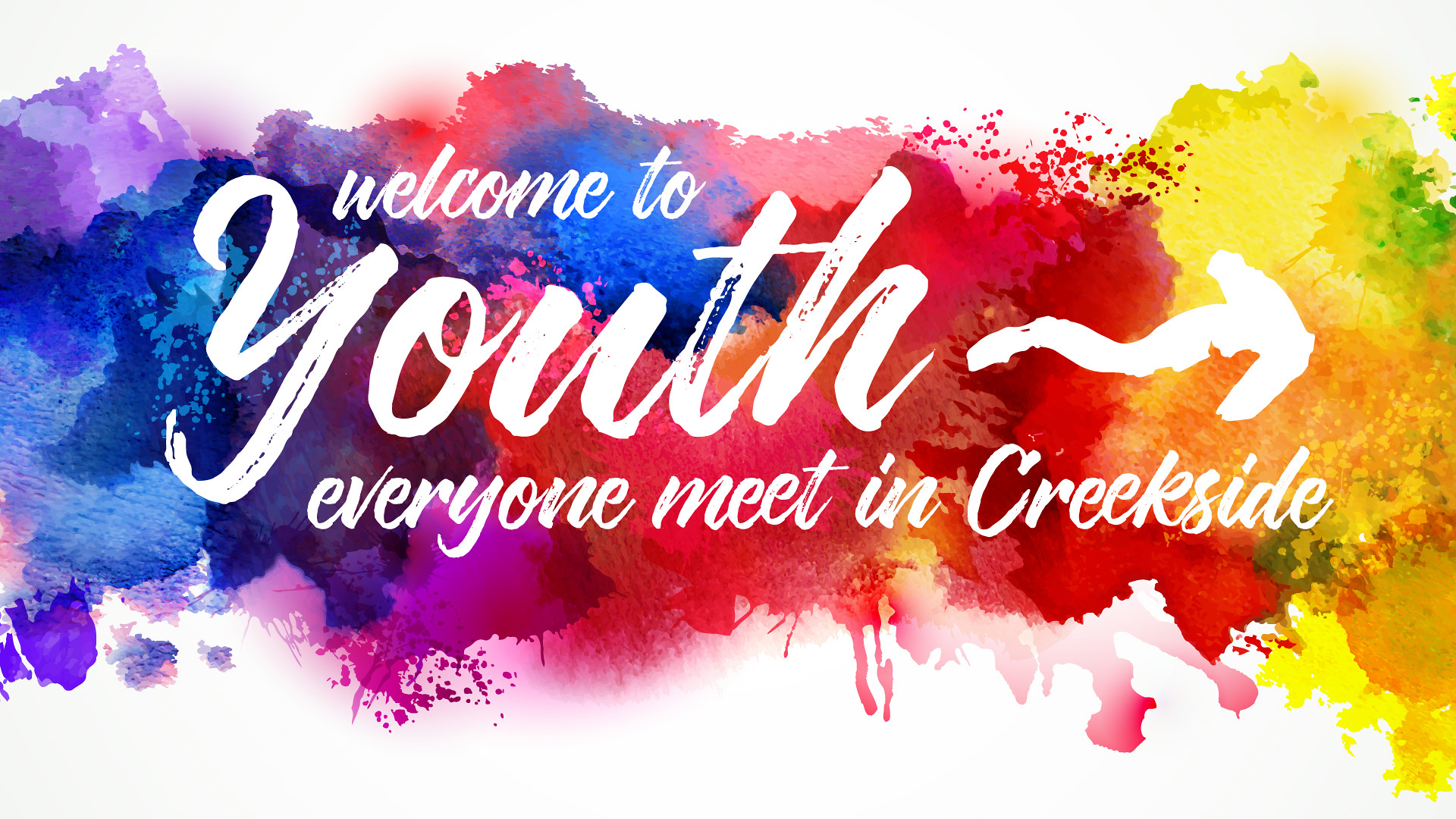The image features a visually striking sign with a solid white background at the top and bottom, and a vibrant splash of watercolor paint in the center. From left to right, the paint splashes display a gradation of colors: purple, blue, red, yellow, orange, and scattered small splashes of green. Overlaying this colorful canvas, the white text appears hand-painted, delivering a welcoming and lively message. The first line reads, "Welcome to," followed by the second line "Youth," written in significantly larger font and centered directly below the first line. To the left of the word "Youth" is a right-facing, curvy arrow. Below this, in smaller text, the third line reads, "Everyone meet in Crickside," also centered. The overall effect combines the spontaneity of paint splashes with neatly arranged, inviting white text, creating what appears to be a digitally created, watercolor-styled advertisement for a youth event in Crickside.